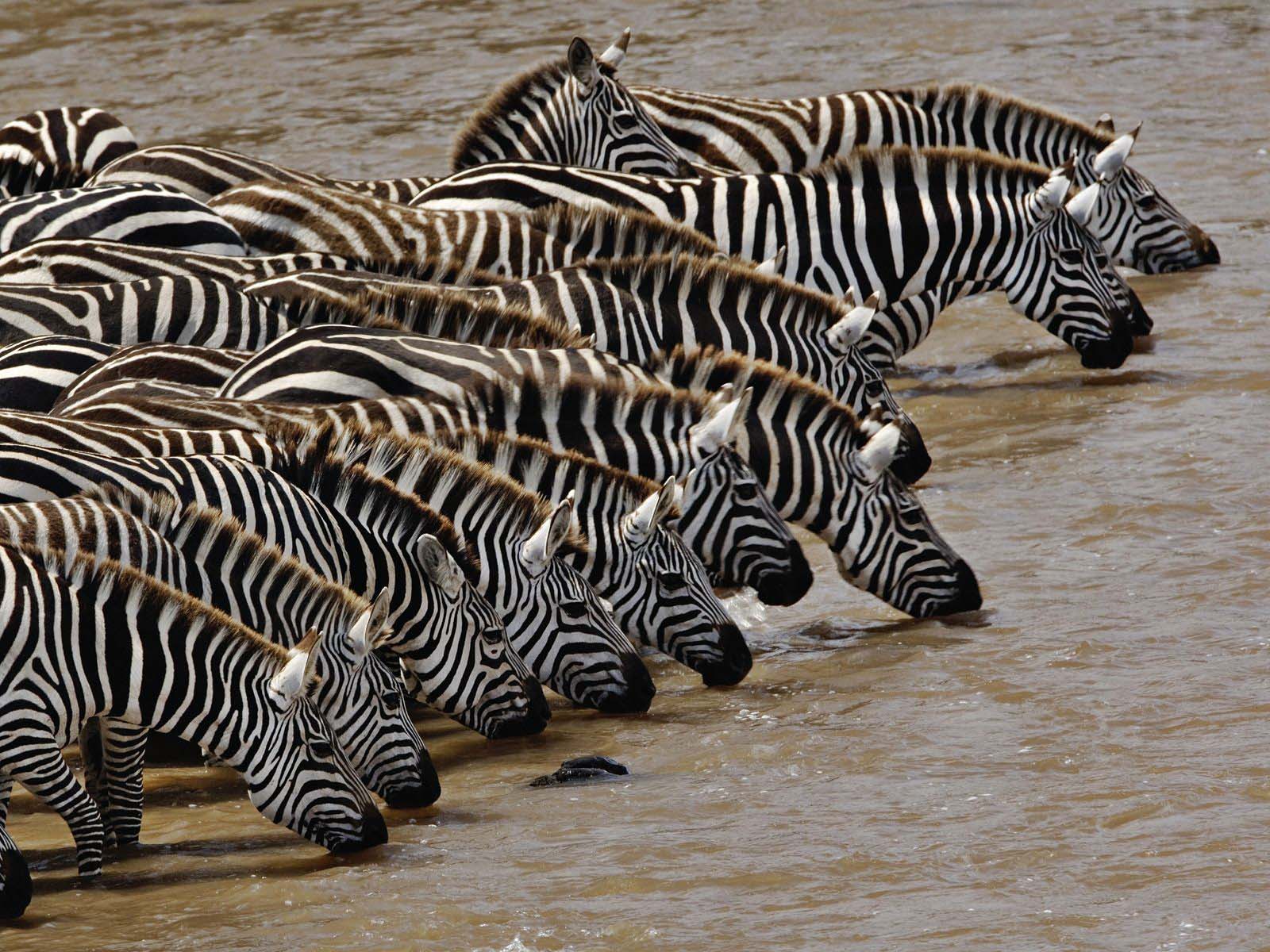In this detailed photograph taken outdoors during the daytime, a herd of approximately 16 zebras is congregated in a shallow, moving body of brownish water, which appears to be a river. The scene is sunlit, suggesting a warm day, with most zebras standing up to their knees in the water, drinking. Nearly all of them have their heads down, mouths in the water, and ears perked forward, displaying the characteristic black and white stripes, some with additional markings such as stripes at the base of the ears or black tips. A single zebra stands apart at the far end, merely observing with its head up, while another seems to have its rear facing the rest of the group. The water is visibly moving, with stones scattered within, and ripples indicating the current, affirming it is less likely to be a pond and more likely a river. No text or words are present in the image.